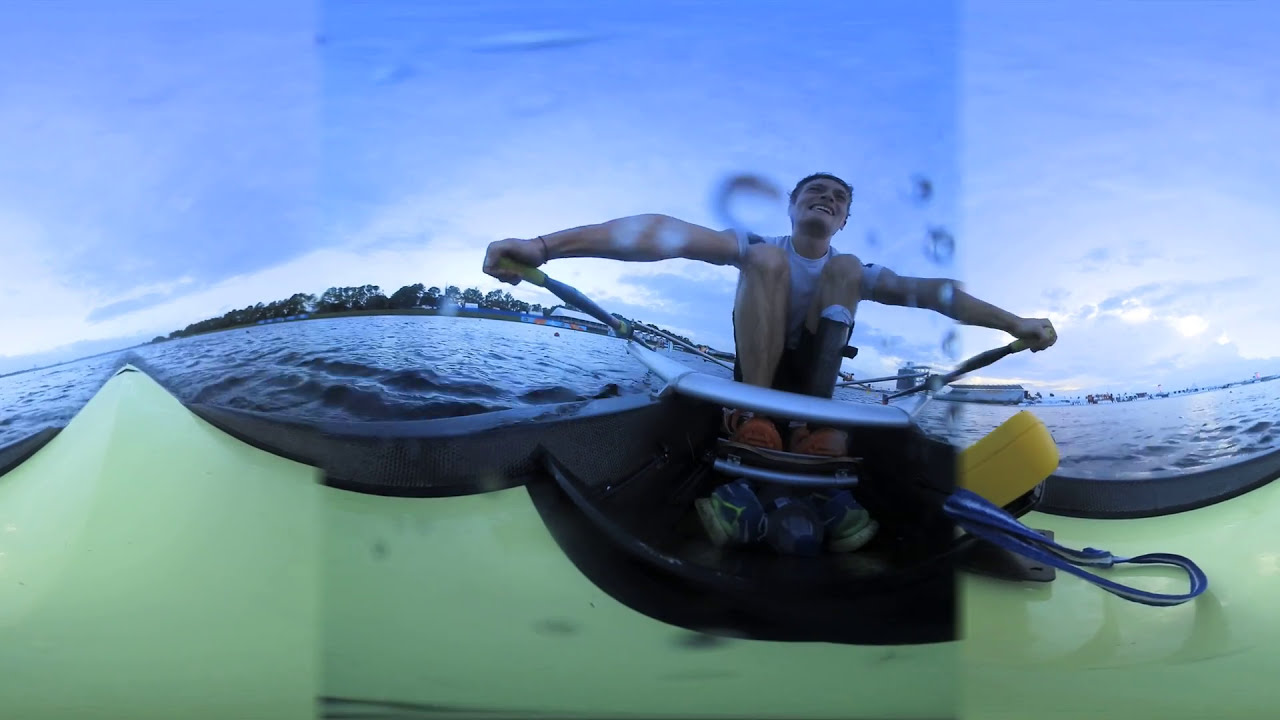The photograph depicts a muscular man kayaking on a large body of water with choppy waves, under a bright blue sky dotted with various white clouds. The man is seated in a bright green kayak, wearing a short-sleeved white t-shirt, black shorts, and orange shoes. He is smiling as he rows, with his arms outstretched, holding two oars. The oars have yellow handles and blue blades. Straps from his kayaking gear are visible, and there is a black object jutting out from the kayak's surface. Water droplets are splattered on the camera lens, suggesting the encounter with the water was dynamic. In the background, a dense line of lush green trees lines the distant land, and there are some buildings visible to the left. The photograph captures a daytime adventure, highlighting the serene yet active environment.